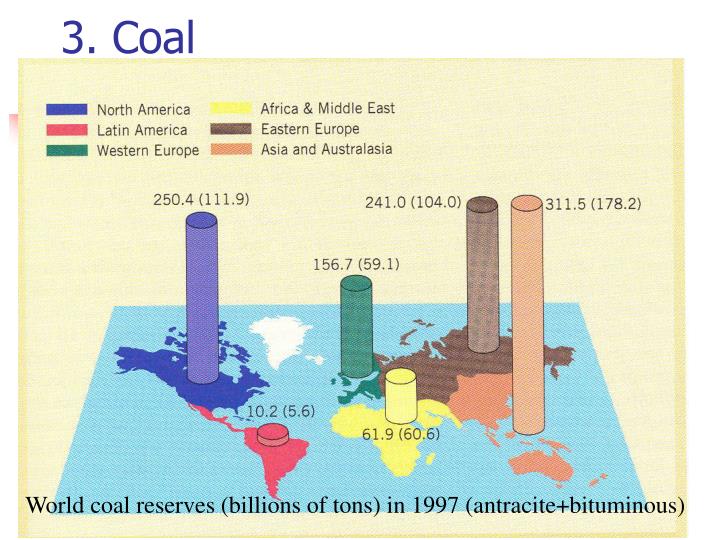This image is a detailed quasi-3D illustration of a bar graph superimposed on a world map, providing a visual representation of global coal reserves in 1997. The map is rectangular and laid out on a tan background, viewed from an upper angle. Each region or continent is color-coded: North America in deep blue, Latin America in red, Western Europe in green, Africa and the Middle East in yellow, Eastern Europe in dark brown, and Asia and Australia in light brown. Emergent cylindrical bars rise from the center of each region, indicating the volume of coal reserves in billions of tons. 

The labeling is clear, with a legend at the top left specifying the regional colors. Above the legend, in large dark blue text, is the number "3" followed by the word "coal."  At the bottom of the image, it states "World Coal Reserves" in black text, followed by "billions of tons in 1997" in parentheses, specifying anthracite and bituminous coal types. Numerical values such as 250 and 156 are present, presumably indicating the quantity of reserves. This image could likely be found in a textbook or an academic presentation, illustrating which regions have the most significant coal reserves.